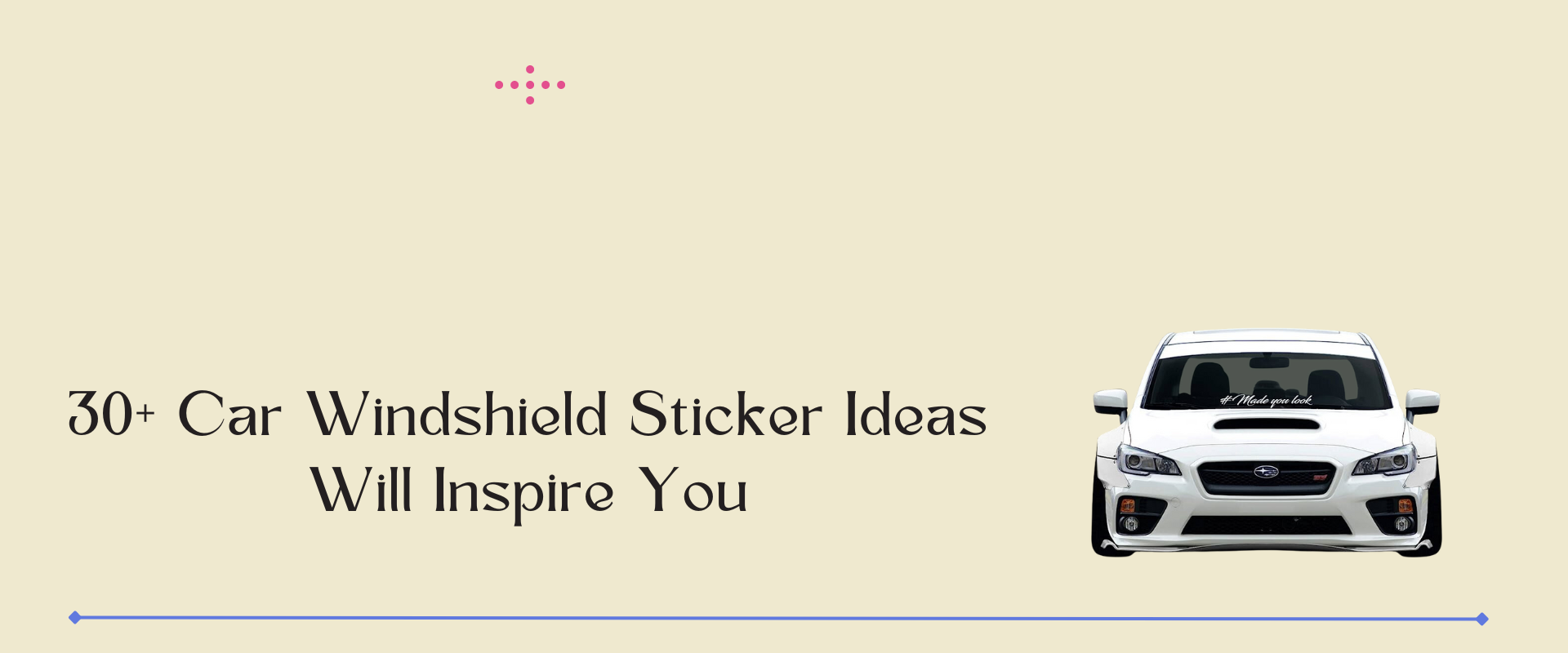The image is a rectangular poster set against a beige background. At the top left corner, there is a red cross made of dots. Below this, in black text, it reads "30 plus car windshield sticker ideas will inspire you." Just beneath this text is a long, thin blue line stretching horizontally across the poster. To the right side of the blue line, there is a detailed drawing of a white sports car, identified as a Subaru by the logo on its grill. The car is depicted from a front view, showcasing its headlights, mirrors, black tires, tire flaps, and black grating on the front hood. The front windshield features an unreadable sticker in white text. The windshield is slightly silhouetted, allowing the car seats inside to be faintly visible.